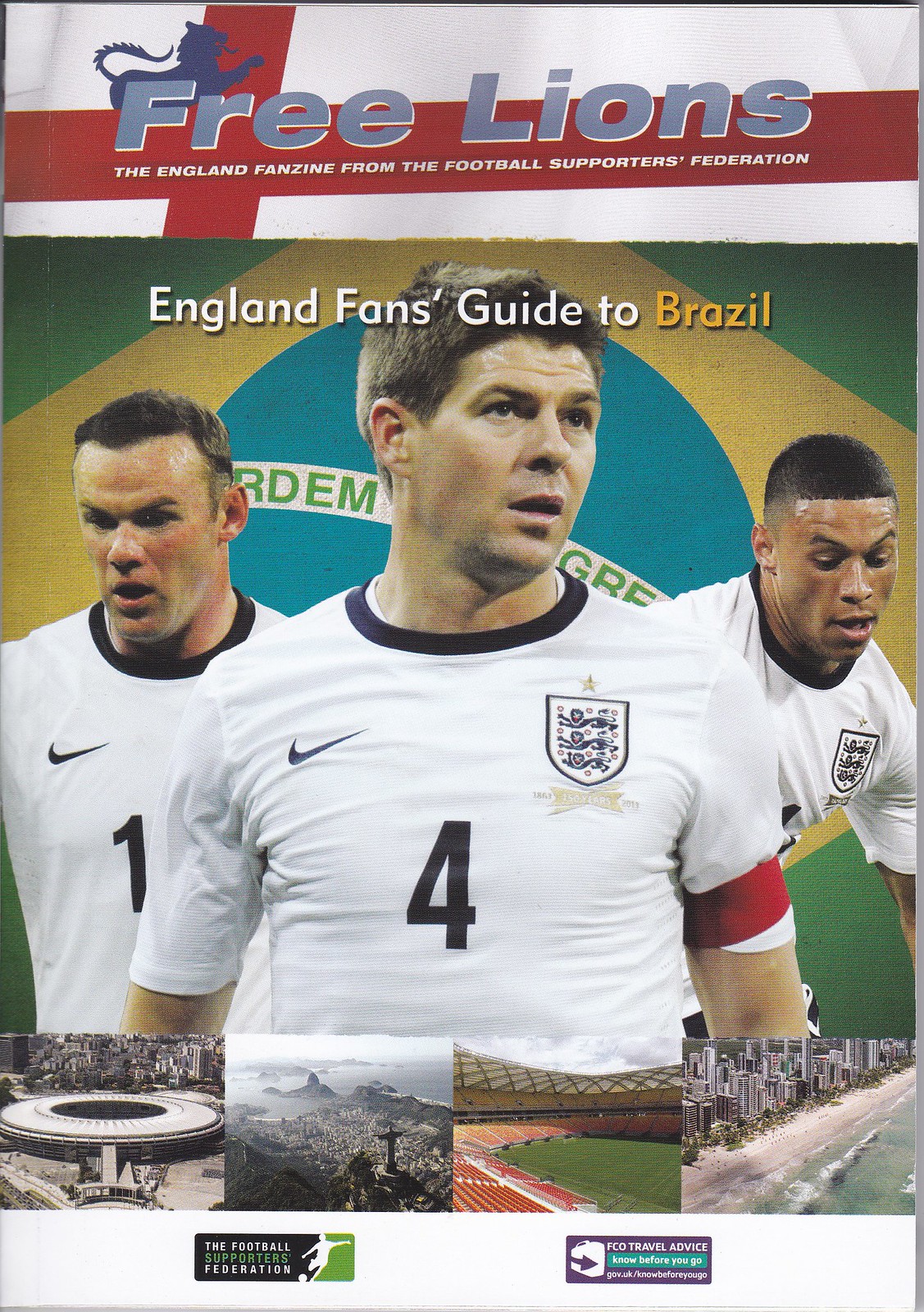The image is a detailed photograph of the front page of a program titled "Free Lions," produced by the Football Supporters Federation for England football fans. The cover prominently features the club's lion logo in the upper left corner, alongside the title. The tagline reads "The England Fanzine from the Football Supporters Federation," with an additional headline, "England Fans Guide to Brazil." The main visual element is a photograph of three men, each wearing a white Nike t-shirt with black collars, adorned with the lion insignia and red armbands. The man in the middle, who is white, wears the number four and gazes slightly away from the camera. To his right, a brown man also in a number four shirt looks downward, while to his left, a white man in a number one shirt looks away. Below this image, there are four smaller photos depicting various scenes: a football stadium, the view from a mountaintop, the stadium stands, and a beach, likely showcasing Brazilian landmarks. At the bottom, there are two logos: one for the Football Supporters Federation featuring a football player graphic, and another for ECO Travel Service with the slogan "Know Before You Go" and a suitcase graphic.